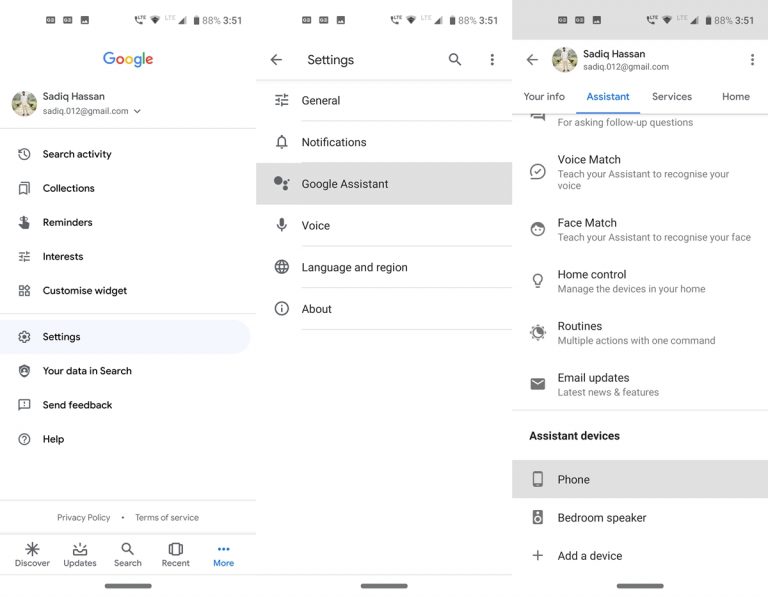In this series of three mobile device screenshots, the user’s interface is displayed with various details highlighted. 

1. **Screenshot 1:**
   - **Status Bar:** The top of the screen shows the Wi-Fi is enabled, LTE network is active with three carrier bars, battery life at 88%, and the time is 3:51 PM.
   - **Profile Section:** There is a profile picture of a man wearing a white shirt and khaki pants, identified as Sadiq Hassan. His email is sadiq.012@gmail.com. A drop-down caret indicates there are additional account options.
   - **Google Services Menu:** The Google icon is visible, followed by menu options including Search activities, Collections, Reminders, Interests, Customize widget, Settings, Your data in Search, Send feedback, and Help.
   - **Navigation Bar:** At the bottom, 'Discover Updates' is shown, 'Search' is highlighted, and there are options for 'Recents' and 'More' available via hyperlinks.

2. **Screenshot 2:**
   - **Settings Navigation:** The user has navigated to the settings tab within the Google app, specifically looking for **Google Assistant** settings.

3. **Screenshot 3:**
   - **Assistant Settings Highlighted:** The focus is on the **Assistant** tab, indicated by bolded text. The section for **Assistant Devices** has **Phone** selected with a greyed-out button in detail.